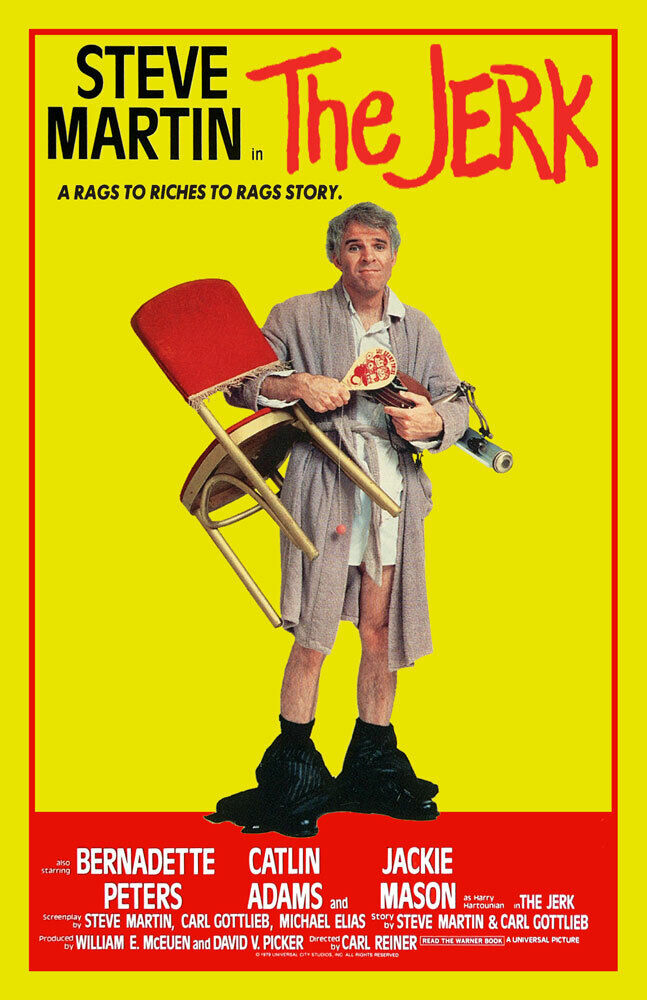This movie poster for "The Jerk" features a bright yellow background with a red border around the central image, fading into a red banner at the bottom. The top left corner of the poster displays the text "Steve Martin in" in black, followed by the title "The Jerk" in bold red letters. Beneath the title, the tagline "A rags to riches to rags story" is written in black.

At the center of the poster is a comical image of Steve Martin. He is depicted in a slovenly manner, wearing a disheveled bathrobe and a white coat or shirt hanging down to his thighs. His gray hair is messy, and his face is scruffy and dirty. Martin comically holds a ping pong paddle in one hand and balances a chair on his arm. His pants are around his knees, revealing black boots, and he appears to be standing in a puddle.

The red banner at the bottom of the poster lists the names of the cast and crew in white text: "Bernadette Peters, Caitlin Adams, Jackie Mason, Steve Martin, Carl Gottlieb, Michael Elias, Steve Martin and Carl Gottlieb, William E. McEwen, David Picker, Carl Reiner."